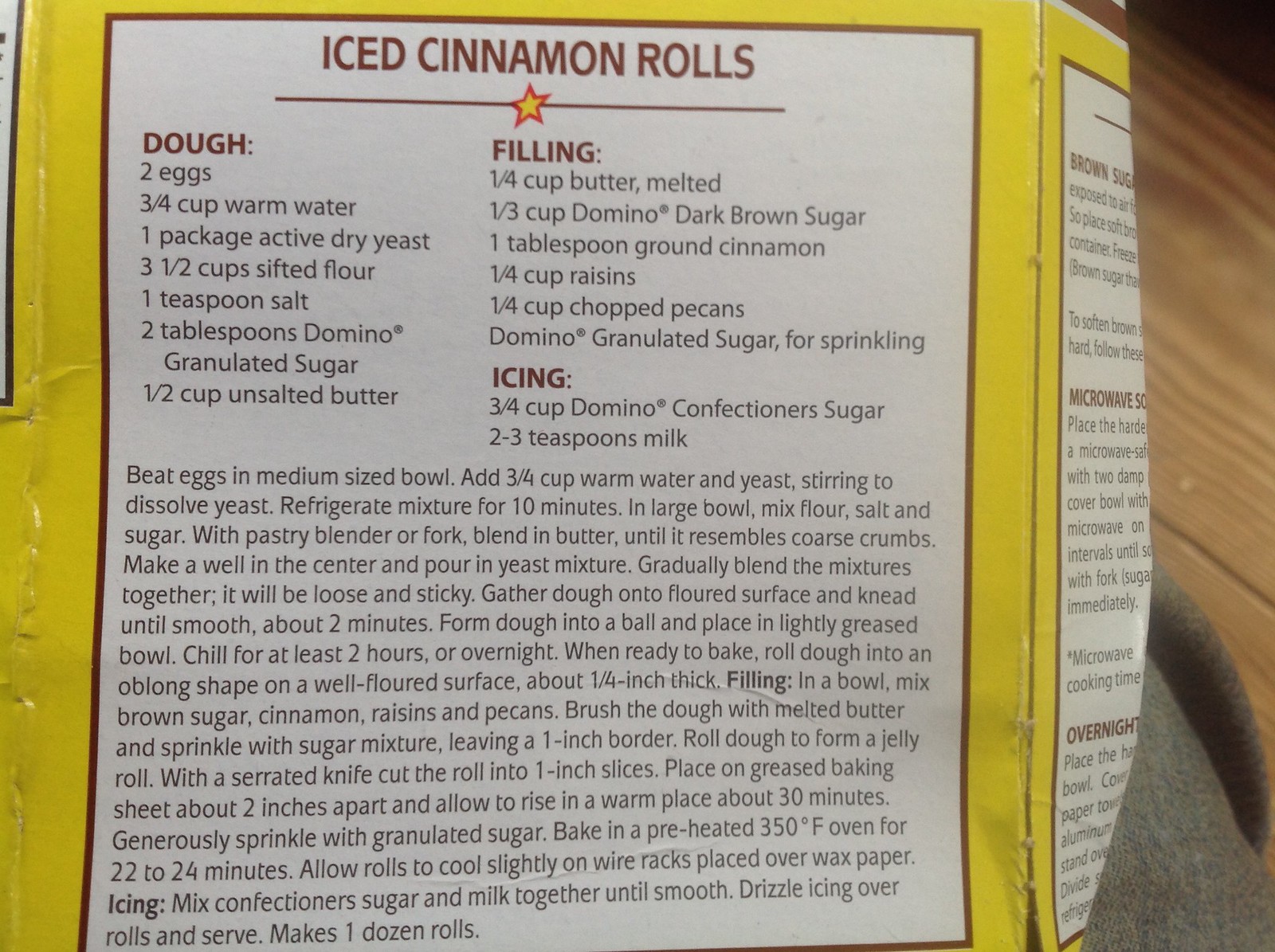The image depicts a close-up view of the back of a yellow Domino Sugar box, which has been slightly smashed on the right side. The box is resting on a surface that appears to be blue jeans, with a wooden floor visible in the background.

The main focus of the image is an extensive recipe for iced cinnamon rolls, presented in brown writing on a white background. Above the recipe, there's a brown line with a gold star below the header "Ice Cinnamon Rolls." The recipe is divided into three sections: dough, filling, and icing. It includes detailed lists of ingredients, such as two eggs, three-fourths cup warm milk, one package of active dry yeast, three-and-a-half cups sifted flour, one teaspoon of salt, two tablespoons of Domino granulated sugar, and one-half cup of unsalted butter for the dough. The filling requires one-fourth cup melted butter, one-third cup Domino dark brown sugar, one tablespoon ground cinnamon, one-fourth cup raisins, and one-fourth cup chopped pecans, with additional Domino granulated sugar for sprinkling. The icing calls for three-fourths cup Domino confectioner's sugar and two to three teaspoons of milk.

Instructions for preparing the dough and assembling the rolls are included, starting with dissolving the yeast in warm water and blending the mixture with flour, salt, sugar, and butter. The dough is then kneaded, chilled, rolled out, filled, sliced, allowed to rise, and baked. The finishing touch involves drizzling the buns with icing after they have cooled slightly.

Additionally, there's some text on the right side related to microwaving brown sugar clumps, although it is partially obscured. The image background shows a neatly composed scene with elements indicating an indoor setting.